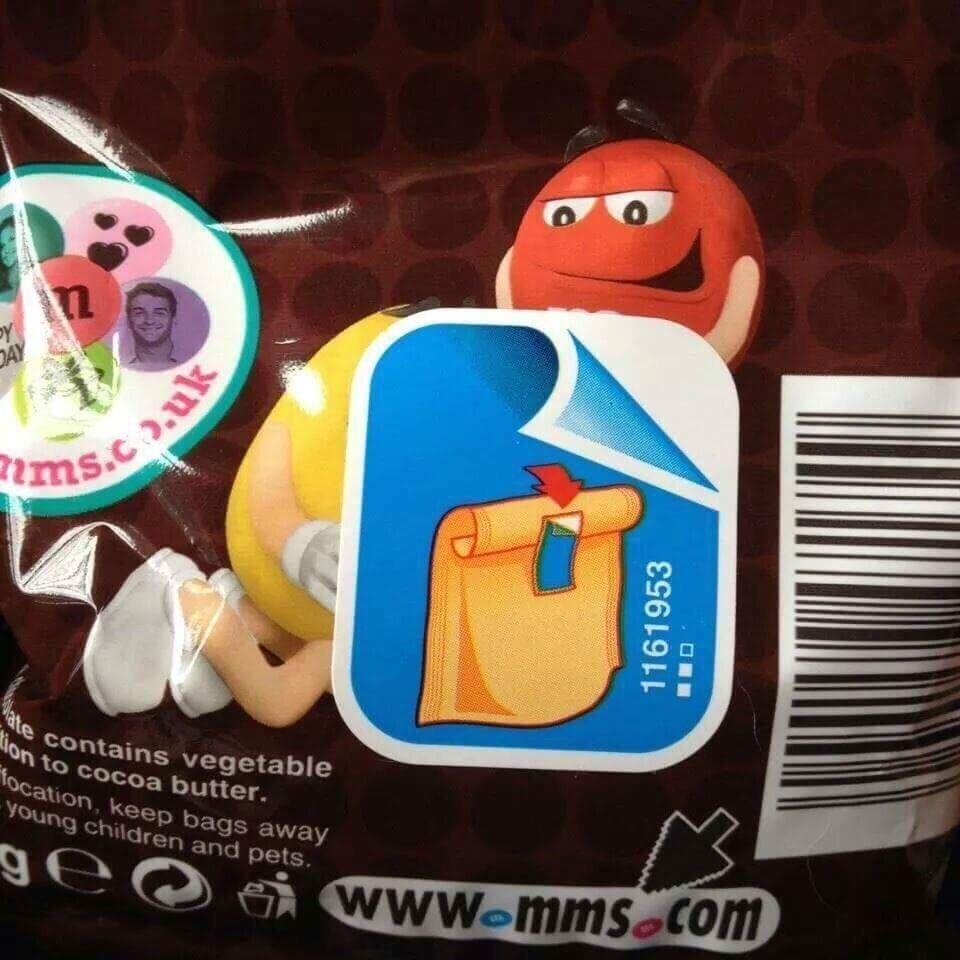The image is a close-up of the back of an M&M's package with a polka dot pattern featuring brown and black circles. Dominating the center-top of the image is the orange M&M character, smiling with expressive eyes, small black ears, and white-gloved arms. Slightly below and to the left of the orange M&M is the yellow M&M, partially obscured by a blue peel-off label; only part of his yellow body, an arm with a white glove, and a leg with white sneakers are visible. 

The blue label intersects both M&M characters and has a torn section revealing a vertical number "1161953" on a white background, alongside an illustration of a rolled-up piece of brown paper with a red arrow pointing at a piece of tape. To the right of this label is a barcode, though the numbers are cut off and only the lines are visible. At the very bottom, the URL "www.mms.com" is displayed in large brown letters.

In the bottom left corner, text appears to inform that the product contains vegetable ingredients and cocoa butter, but part of this text isn't fully visible. Additionally, warnings about suffocation and keeping the bag away from young children and pets are partially legible. There are also various icons and logos at the bottom, though they aren't clearly defined.

In summary, this detailed description captures the key visual elements from the captions, focusing on the main features and shared observations about the back of the M&M's package.